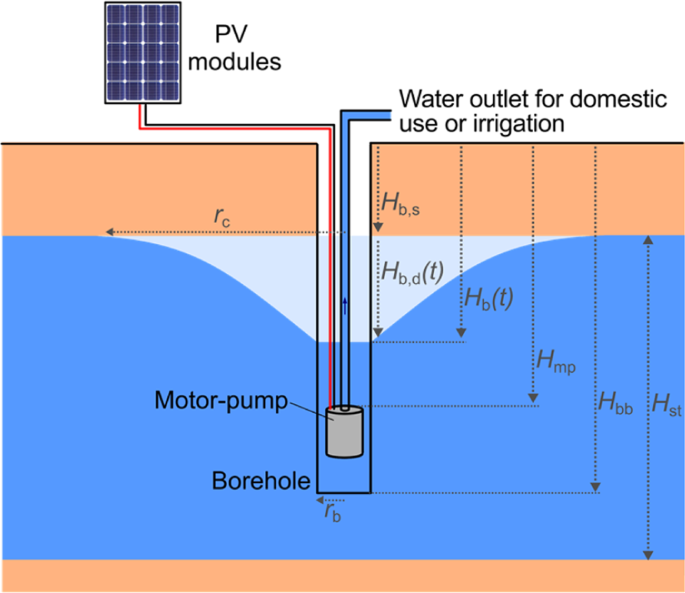This image is a detailed, digitally created diagram illustrating a solar-powered irrigation system. In the top left corner, labeled in black Arial font, are the "PV modules," depicted as solar panels. From the PV modules, red and black lines extend downward and then to the right, connecting to a gray cylinder labeled "motor pump," which appears buried underground. This motor pump connects through a blue pipe that extends rightward above the ground, terminating at the "water outlet for domestic use or irrigation." The diagram's background features a top strip of beige, representing the earth's surface, followed by a large blue section indicating underground water. Beneath this blue section, there's another thin strip of beige, symbolizing further ground layers. Several labels with subscripts (HBS, HBDT, HBT, HMP, HBB, HST, RB, RC) on the right side indicate different heights from the surface to various levels of the system, marked by corresponding arrows. Overall, this chart details the process and components involved in drawing water from an underground borehole using a solar-powered motor pump for irrigation or domestic purposes.